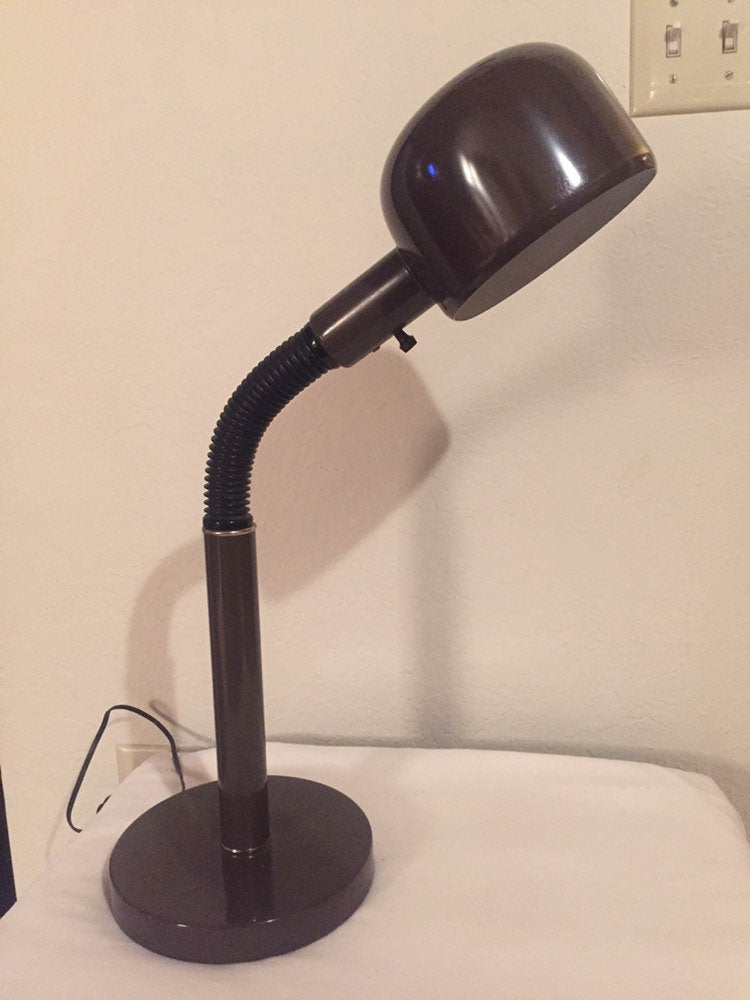In the portrait-oriented image, a sleek black desk lamp stands prominently on a small, white rectangular table. The lamp, featuring a shiny, rounded base, transitions into a ribbed, bendable neck that adjusts the light direction. The top of the lamp ends in a deep bowl-shaped dome with a switch beneath for easy operation. This black lamp is positioned against a beige wall that casts its shadow, adding depth to the setting. The wall also includes a light switch panel in the upper right corner, housing two white switches. An electrical cord extends from the lamp's base, trailing behind the table and connecting to a partially visible outlet. The tabletop appears to be covered with some fabric, possibly a cloth or a shirt, adding a subtle texture to the scene.